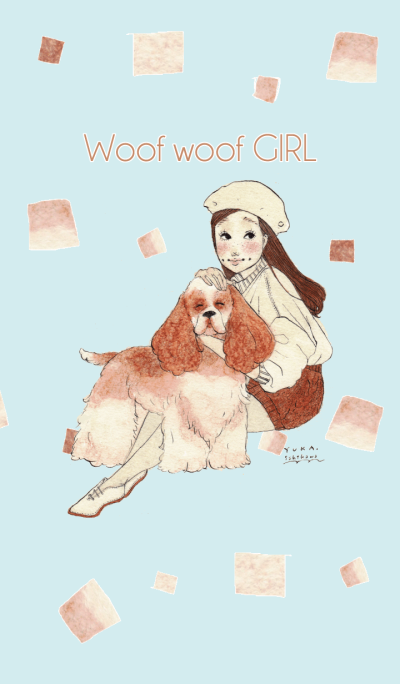This is a detailed illustration captured on a poster titled "Woof! Woof! Girl" written in light brown, capital letters on a predominantly turquoise background. The central figure is a young girl with brown hair, blushing cheeks, and dressed in a cream beret, a matching cream sweater, and brown shorts. She is lovingly hugging a fluffy cocker spaniel with large brown ears; her right hand rests gently on the dog's head and her left hand under its neck. The dog's eyes are closed in contentment as it stands over her outstretched legs, revealed under the dog, adorned with small white shoes. Above the girl, the sky is filled with various sized squares in brown and white, resembling either marshmallows or sugar cubes, cascading down gently. The overall scene embodies warmth and companionship between the girl and her happy spaniel.